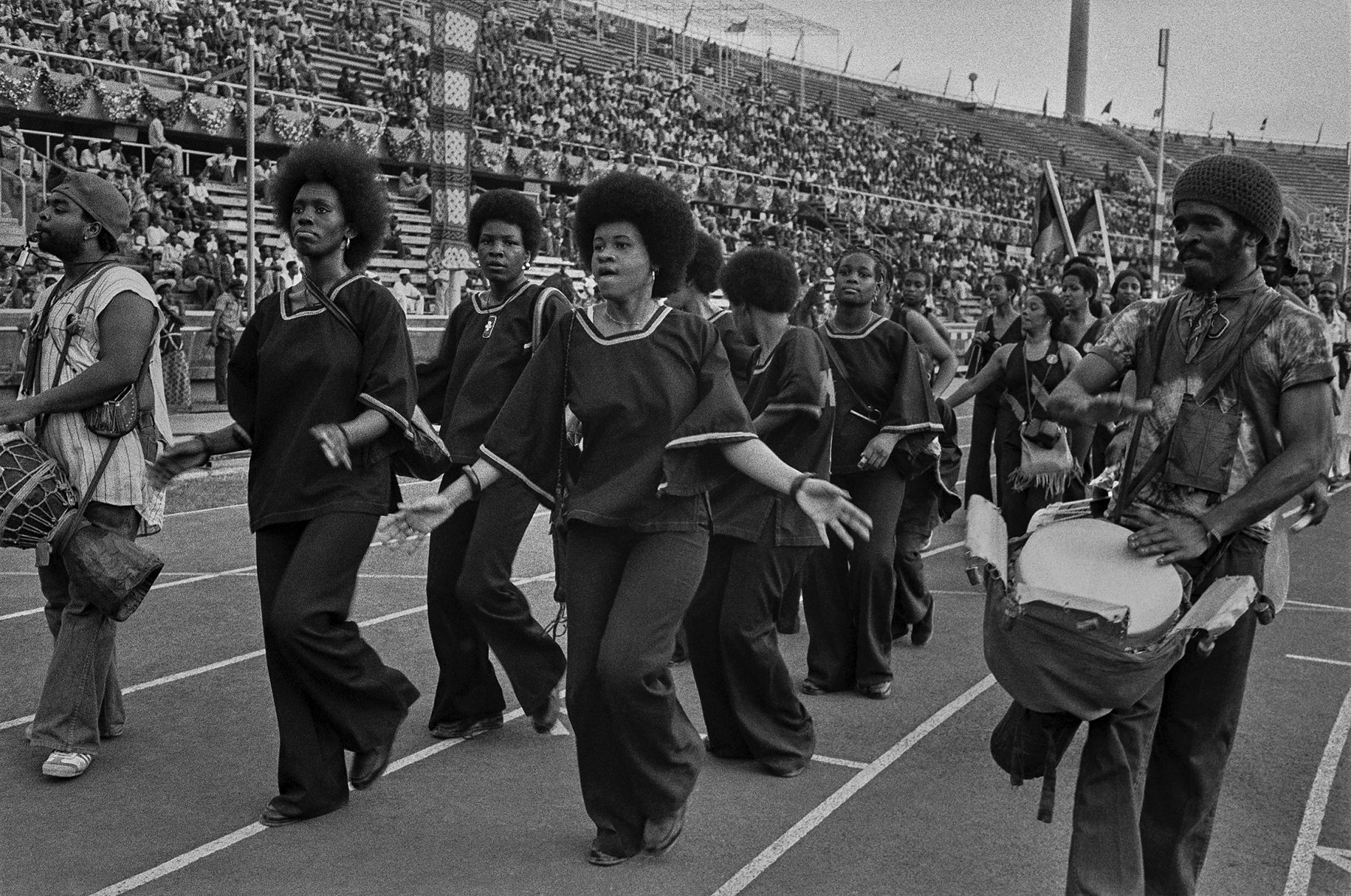This vintage black-and-white photograph from the 1960s captures a lively parade scene inside a crowded stadium, possibly in the United States. The image showcases African American performers in vibrant action. Central to the photograph are female performers with large 1960s-style afros, dressed in coordinated costumes, who appear to be singing and dancing energetically. They are flanked by two male drummers, one on each side; the drummer on the right is identifiable by his knit cap and beard, while the drummer on the left stands equally prominent. In the background, a throng of participants can be seen carrying flags and wearing various outfits, contributing to the festive atmosphere. The stadium bleachers are filled to the brim with spectators, highlighting the sizable crowd and adding to the celebratory ambiance of the event. A person with shoulder strap bags stands in the forefront, possibly carrying supplies for the participants. The detailed capture encapsulates a moment of cultural expression and community gathering, characteristic of the era.